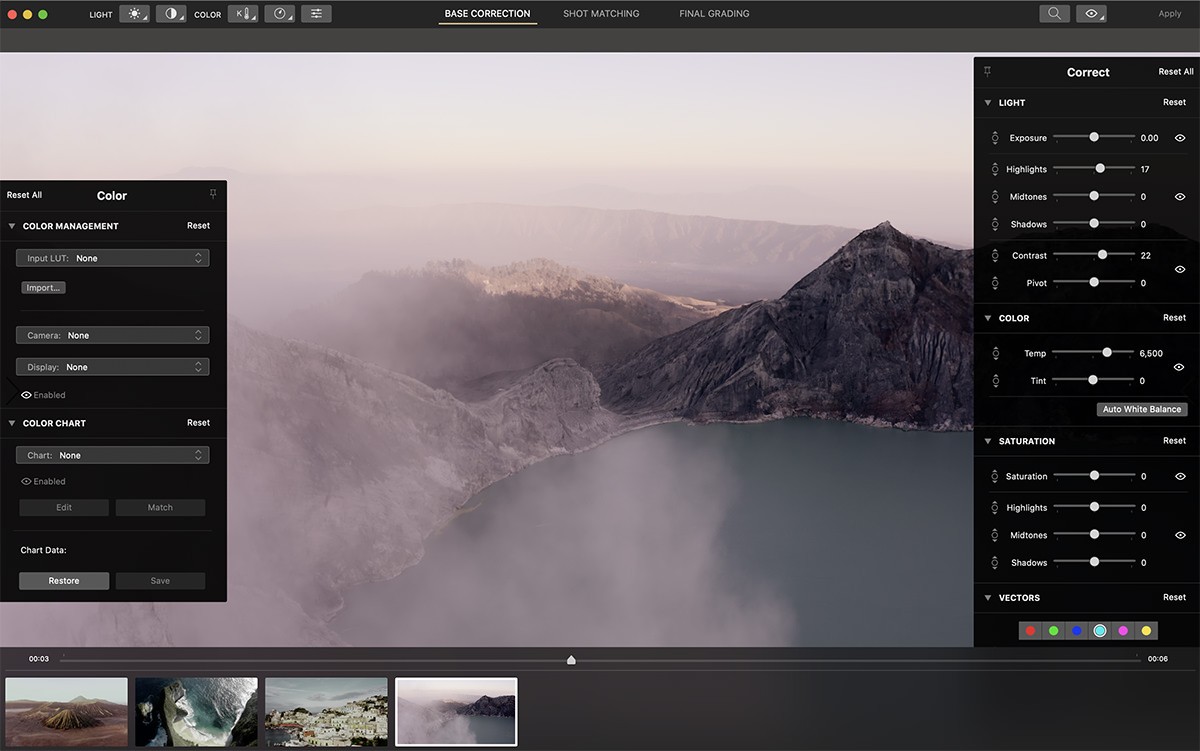The image is divided into several segments, displaying a detailed interface of a color grading application. The bottom four images depict various natural landscapes: one of a mountainous region, another showcasing an ocean region, a snowy mountain scene, and a foggy lake. 

In the top-left corner, there are red, yellow, and green indicators. Next to these indicators is a gray square with a sun symbol, potentially representing brightness or exposure settings. Adjacent to it, there are settings labeled like “Base Correction,” “Shot Matching,” and “Final Grading,” presumably steps in the color correction process.

To the far left, various tools related to color management are presented, such as “Color,” “Camera,” “Display,” and “Color Chart.” These tools assist in adjusting the overall look and feel of the images.

On the right side of the interface, there are multiple correction tools: “Reset All,” “Lights Reset,” “Exposure,” “Highlights,” “Midtones,” “Shadows,” “Contrast,” and “Saturation.” Each of these settings allows detailed adjustments to different aspects of image color and light dynamics. Underneath these settings are additional fine-tuning options for highlights, midtones, shadows, and vectors, ensuring precise control over the image colors.

Below, a color spectrum bar includes red, green, blue, light blue, purple, and yellow colors with corresponding eyeball icons, likely used for visual confirmation or toggling layers in the editing process.

In the center, a prominent image showcases a foggy, misty landscape with mountains and coastal hedges, demonstrating the focus area for the applied adjustments.